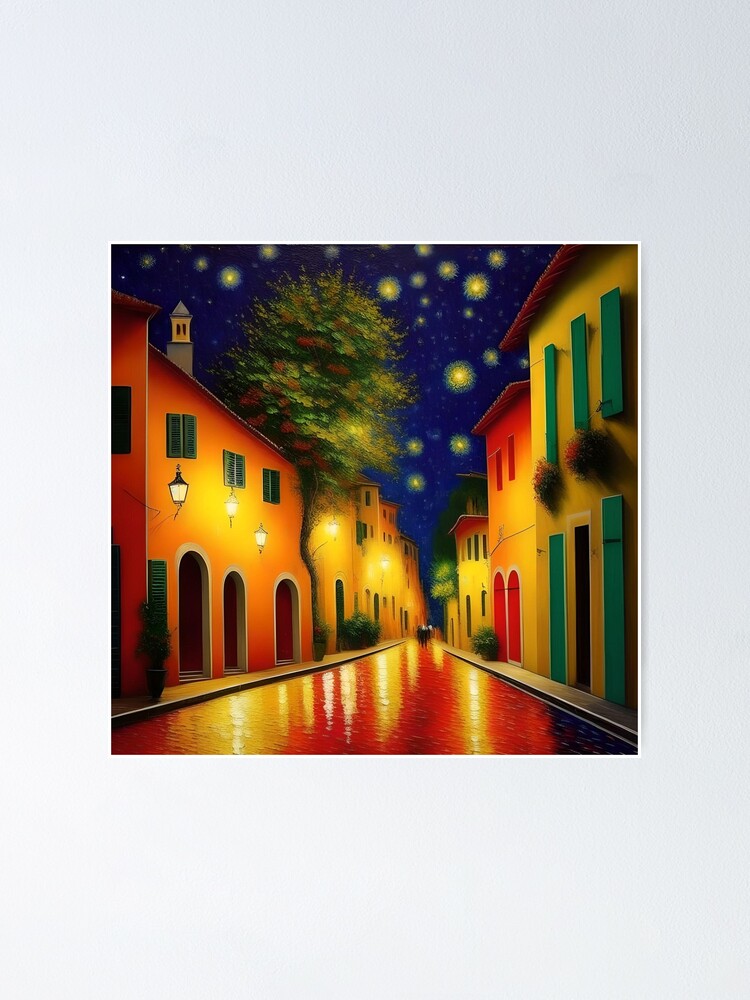The painting, reminiscent of Van Gogh’s style, depicts an idyllic village street scene at night. The street, which runs down the center, almost appears reflective, like a canal in Venice. The village is bathed in vivid colors, with buildings lining both sides of the street. On the left, there's an orange building with archway doors, illuminated by lights hanging from windows. Above this building, a fuzzy green tree with red flowers blends into the scene. The right side features a series of yellow, two-story houses, with the closest house displaying green shutters and a red roof. These houses have distinguishable colored shutters, adding charm to the rustic setting. The vibrant blue night sky above is dotted with golden, star-like balls of light resembling fireworks, casting a warm glow. Additional plant details include bushes along the sidewalks and hanging plants from some windows. At the far end of the street, people are visible, walking towards the viewer, adding a touch of life to the serene village tableau.